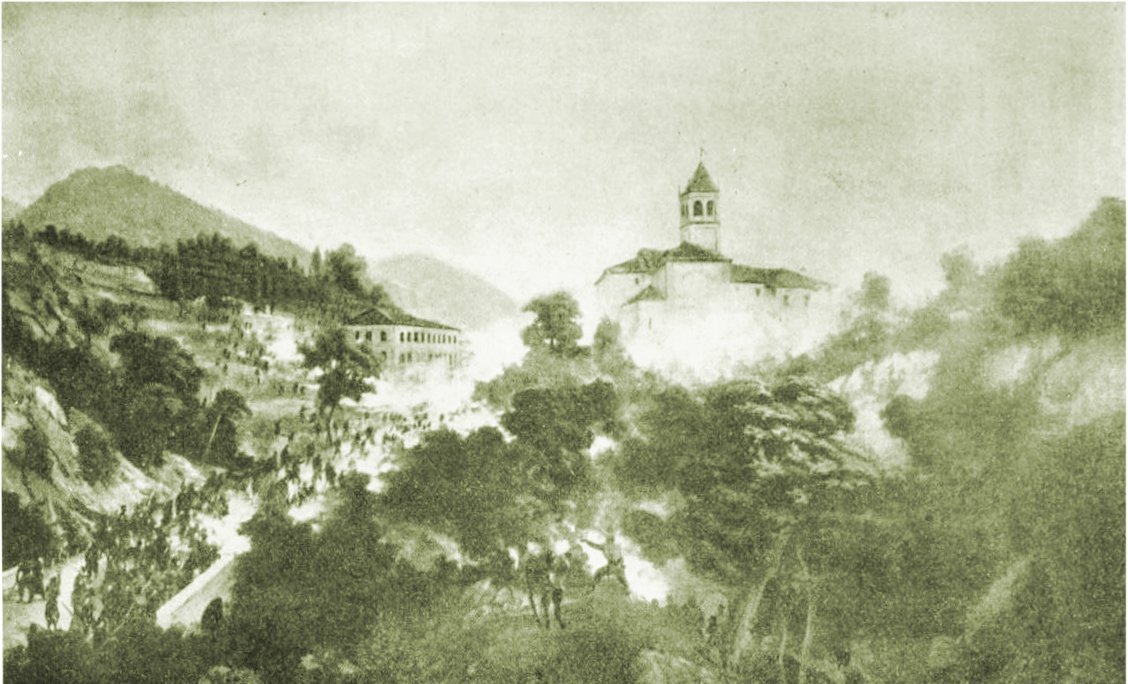In sepia tones, this image—likely a photograph though possibly a painting—depicts a muted, impressionistic landscape on a cold, misty morning. The scene is framed by mountainous terrains on both the left and right sides, rising high against a gray sky. Between these mountains, the top of a building with a steeple is faintly visible, possibly a church or a grand home with a lookout tower. Another building sits to the left, resembling a long hall or barracks with multiple windows and a dark roof. 

The foreground reveals a forested area, seen from above, with dense, richly colored tree canopies shrouded in fog or snow, retreating into a white, illuminated path. Small, distant figures appear to be ascending this path. The overall mood is one of a hazy, detailed autumn or winter day, tinged with greenish-gray hues, giving the entire scene a nostalgic, aged feel.